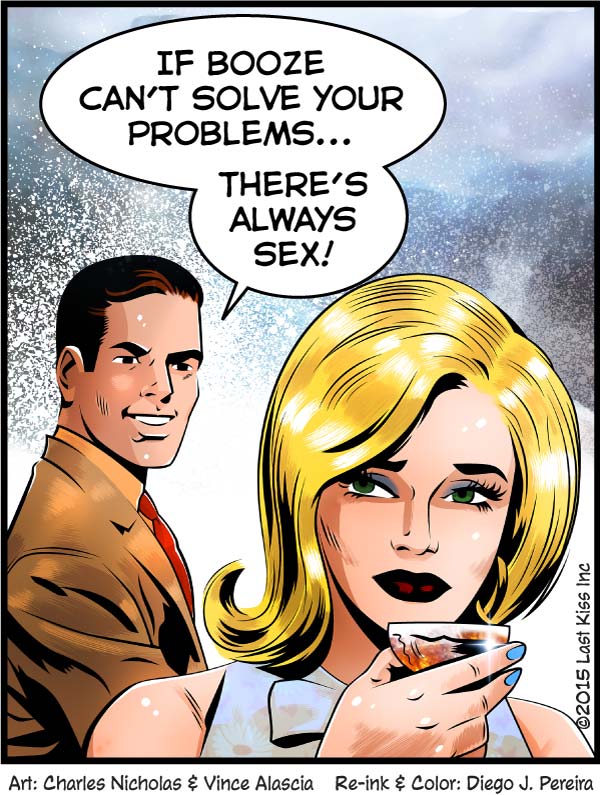In this comic panel, a Caucasian man with short, slicked-back brown hair stands on the left, wearing a brown suit coat, a brown collared shirt, and a red tie. He delivers a statement in a speech bubble above him that reads, "If booze can't solve your problems, there's always sex," with a somewhat malicious expression. To his right, a blonde woman with curly, glowing hair, adorned with blue fingernail polish, is shown from the shoulders up. She holds a martini glass with a brown liquid, has vibrant red lips, green eyes, and wears purple eyeshadow. Her expression conveys annoyance and perplexity at the man's comment. The background is light blue, and the bottom corner of the panel contains credits: "Art Charles Nichols and Vince Alessia," "Re-ink and color Diego Perina," and "2015 Last Kiss Incorporated."